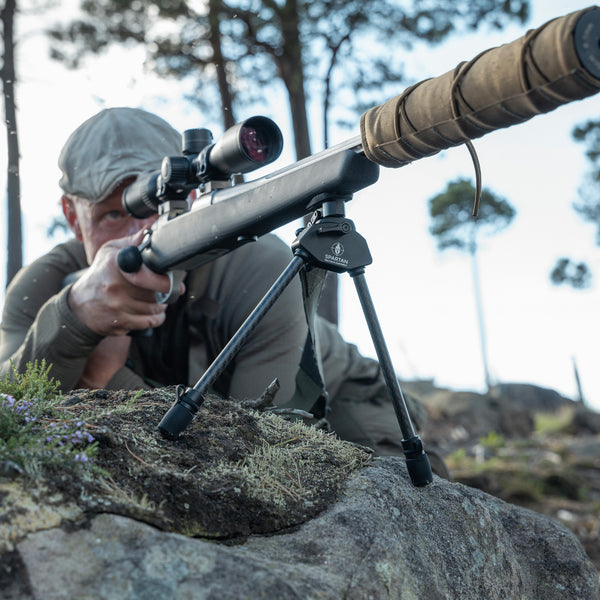In this vivid daytime photograph, a soldier is shown in a focused, sniping position. The man, who is likely in the army, is kneeling or lying down with one eye peering through the large black scope of a sniper rifle. He wears a tan or green hat, along with green fatigues or a tan jacket. The rifle, which is supported by a black tripod for stability, has a long barrel wrapped in a light green or canvas material, camouflaging it against the natural surroundings. The soldier's finger is poised on the trigger, ready for action. He is situated on a gray rock that has patches of foliage, and the backdrop includes rocky terrain and a variety of trees under a lit-up sky. The overall scene captures the tension and readiness of a military operative in the field.